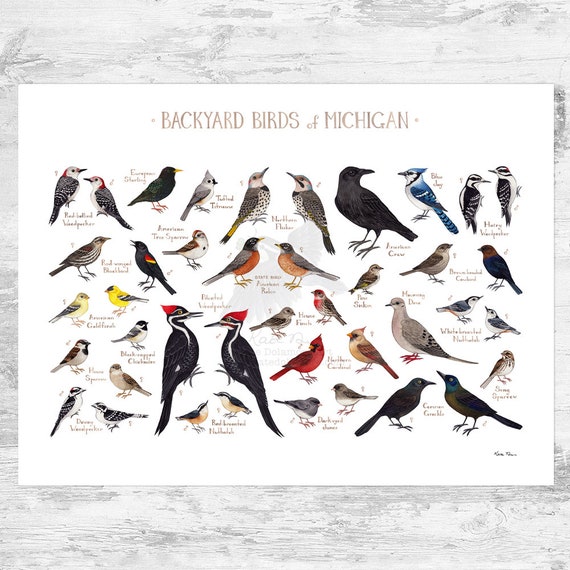The image is a white poster titled "Backyard Birds of Michigan" in light red or gray capital letters at the top. It features a detailed and colorful array of hand-drawn birds spread across the center, with each bird labeled in small print. The birds are organized mostly in rows, though they become more scattered towards the bottom. Notable birds include a blue jay labeled on the top right, crows, cardinals, robins, woodpeckers with red heads, and various small birds in colors ranging from yellow, black, white, red, brown, and green. The background of the image is a light gray, possibly wooden surface, and there's small hard-to-read text in the bottom right corner, which indicates image compression and enlargement from a smaller original.